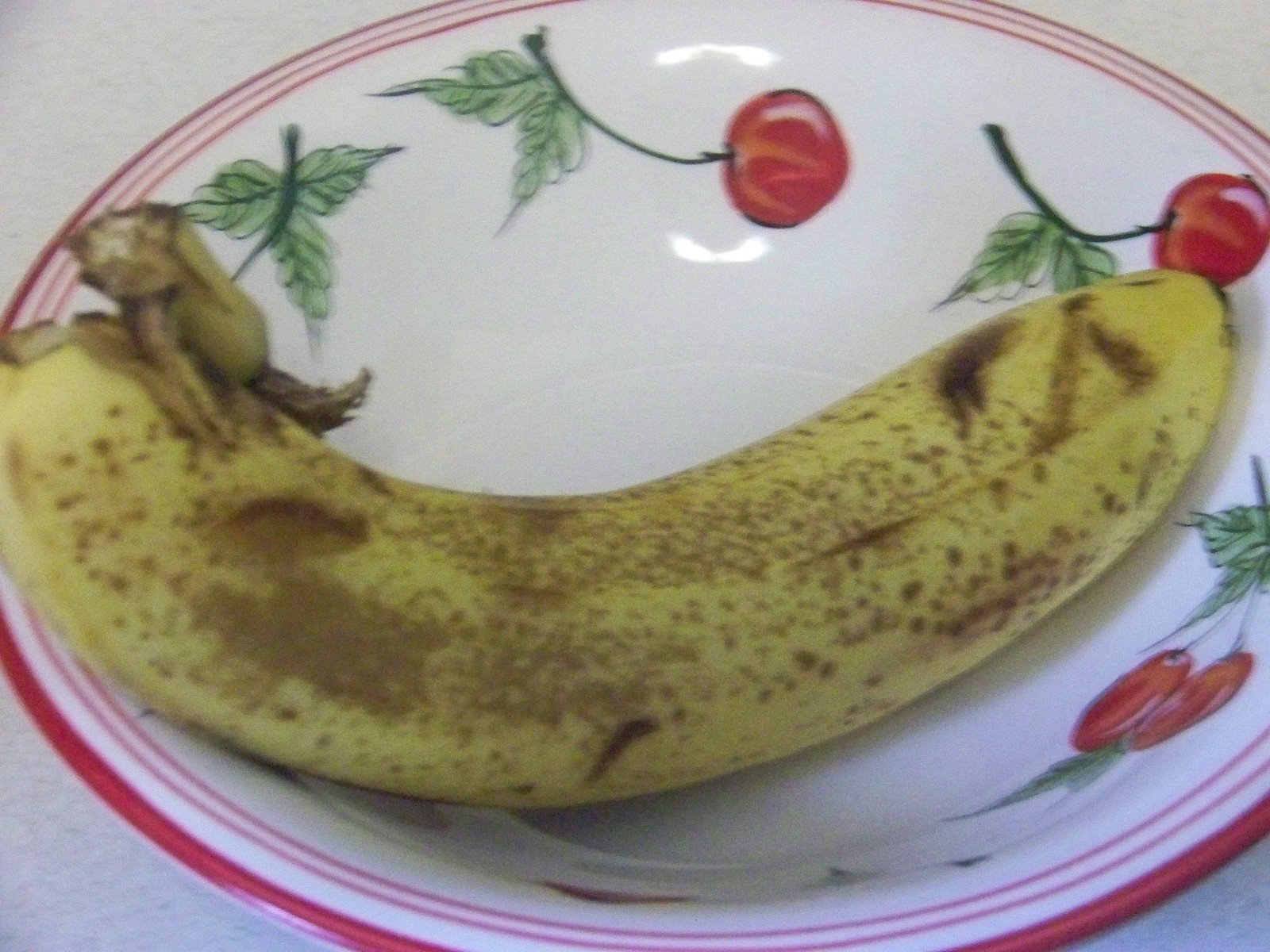A slightly out-of-focus photograph features a ripe banana resting on a shallow bowl. The banana displays a yellow skin with light brown spots, indicating it is ripe. Its stem, partially broken, leans downwards but remains unpeeled. The shallow bowl, primarily white ceramic, is adorned with three red stripes around its rim, interspersed with the white ceramic. Just below the rim, painted shapes resembling either tomatoes or cherries with green stems and leaves encircle the bowl's perimeter. The bowl is set against a light-colored surface, likely a table or countertop, which forms the indistinct background of the image.